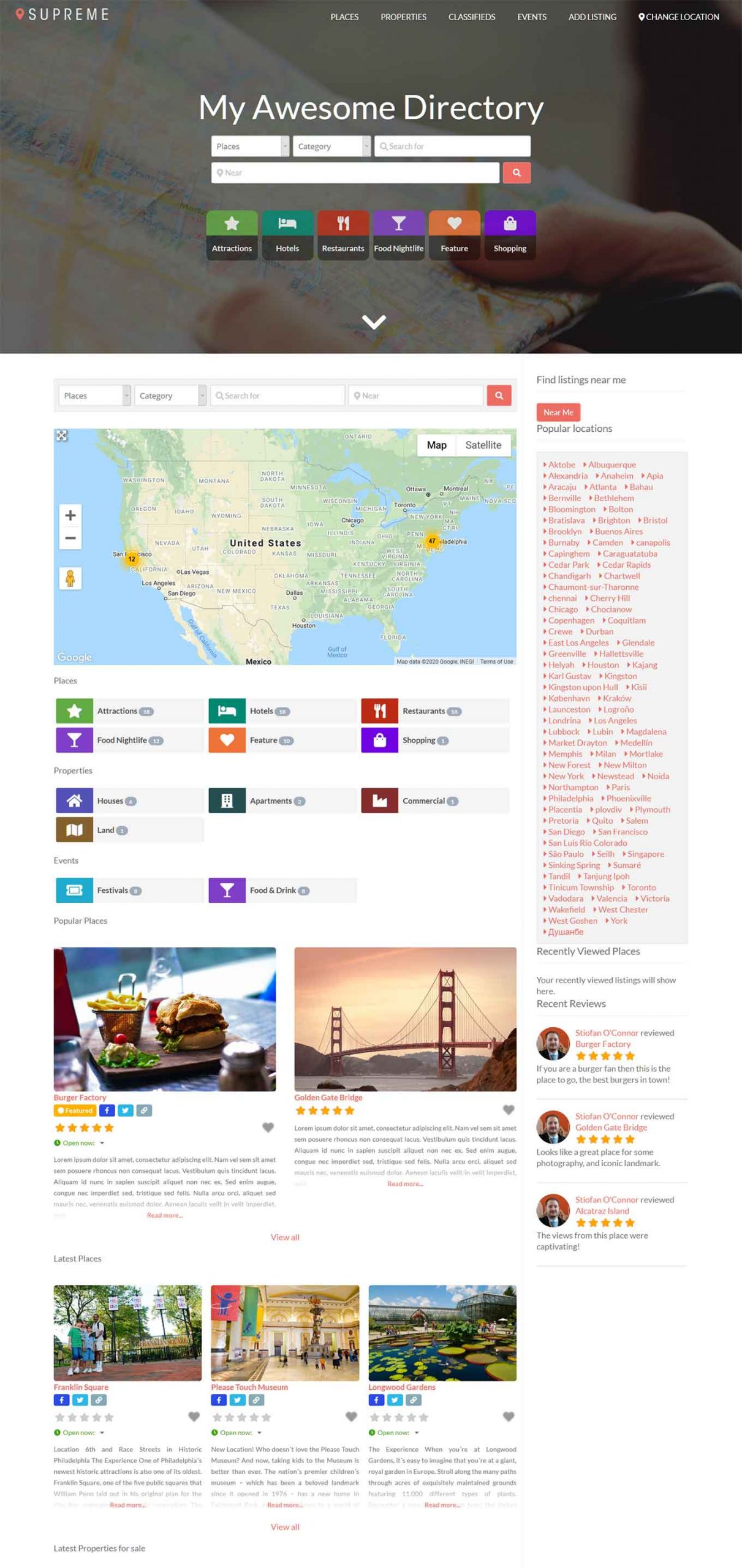This image is a detailed screenshot divided into several sections. 

The uppermost section is in landscape mode and features a "Supreme" logo in the upper left corner. Starting from the top center, the interface includes tabs labeled "Places," "Properties," "Classified," "Events," "Add Listing," and "Change Location."

In the central section, there is a form titled "My Awesome Directory." This form includes various fields such as a dropdown for selecting a category from "Places," a search bar for specific queries, an input for "Next Location" and "Near Location," followed by a prominent red "Search" button. Below this, there are six selection options: "Attractions," "Hotels," "Restaurants," "Food," "Nightlife," "Feature," and "Shopping." Faintly in the background, there is an image of a person's right hand, with their thumb and finger holding a physical paper map.

The next section displays another screenshot. On the left, similar to the previous form, it contains fields for "Places," "Category," "Search for," and a red "Search" button. Adjacent to this, there is a large map of the United States. Notably, on the left side of the map, there is a highlighted circle with the number "12" near what appears to be San Francisco, and another circle with the number "47" possibly near Philadelphia. The map is further populated with numerous comments regarding various places to stay.

Overall, the screenshot captures a user-friendly directory interface designed to help users search and explore different locations and categories of interest.